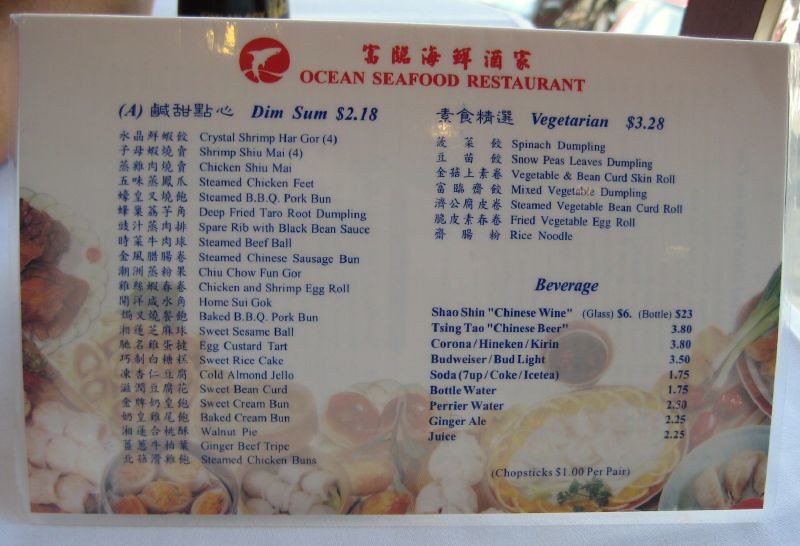The menu board of Ocean Seafood Restaurant is prominently displayed on a wall, affixed to tan-colored 2x4 wooden supports. It occupies nearly the entire image, with only a narrow strip of the background visible at the top. The menu has a cream-colored background. At the top, Asian characters in red script introduce the menu, followed by the restaurant's name in English, "Ocean Seafood Restaurant." To the left of the name, a red circle features a white fish—either a dolphin or a tuna—leaping out of the water.

The menu is divided into two distinct columns. The left column is headed by “Dim Sum – $2.18” in dark blue text, followed by a list of various dim sum options, also in dark blue. The right column features two sections. The upper section is labeled “Vegetarian – $3.28” in dark blue and details the restaurant’s vegetarian offerings. Below it, the “Beverage” section enumerates an assortment of drinks, including both beer and wine. At the very bottom right corner, the menu mentions “Chopsticks – $1.00 per pair” in dark blue text. The bottom of the menu is subtly decorated with faint images of Asian dishes, adding a muted yet elegant touch to the overall design.